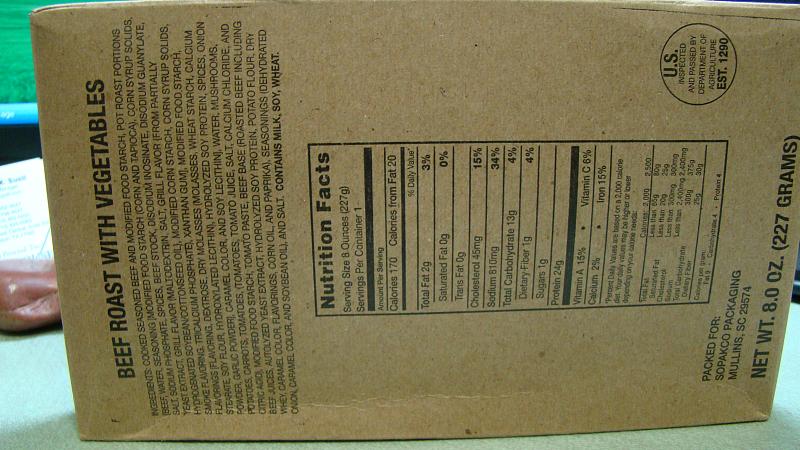This image showcases the back of a beef roast packaging, made from cardboard and oriented horizontally with the top of the package toward the left. To read the text correctly, one would need to turn their head to the left. The prominent black lettering indicates "Beef Roast with Vegetables." A large section below this title lists a comprehensive array of ingredients. Underneath the ingredients, there is a detailed nutrition facts chart displaying various nutrients such as fat, cholesterol, sodium, and carbohydrates. The bottom portion of the package reveals the distributor's information and confirms that the product weighs 8 ounces. On the right side of the packaging, there's a U.S. approval seal, likely related to packaging and handling safety, although the specific details are not entirely legible.